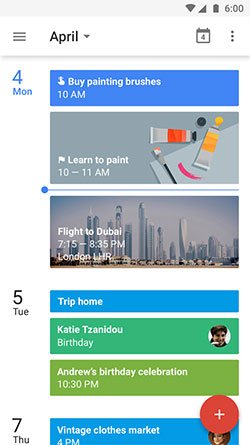### Detailed Caption

In the upper right corner of the screen, the status bar indicates full Wi-Fi signal, full cellular signal, and a fully charged battery, with the current time displaying 6:00. Below the status bar, there's a hamburger menu icon and the text "Dex is this April", alongside a calendar icon.

The calendar interface is now visible, showing different events stacked vertically. Beside each event, a blue tick mark indicates their status. The fourth event of the day is highlighted in blue and titled "My Paintbrush" scheduled at 10:00 AM. Another event, also at 10:00 AM, labeled "Learn to Paint" is noted in grey.

There is an illustration of a paint tube adjacent to these entries, depicting yellow paint coming out of a tube, resembling a paintbrush with a black handle.

Below these events, an informational bar appears, which seems to represent a timeline or a different section. White text indicates that a flight to Dubai is scheduled from 7:15 PM to 8:35 PM, departing from London Heathrow Airport (LHR) with the flight number 523.

Upcoming events and reminders include a trip labeled "Tripp Hall" in blue and birthdays: Katy Tansy Doll and Andrew's birthday celebration from 10:00 AM to 3:00 PM.